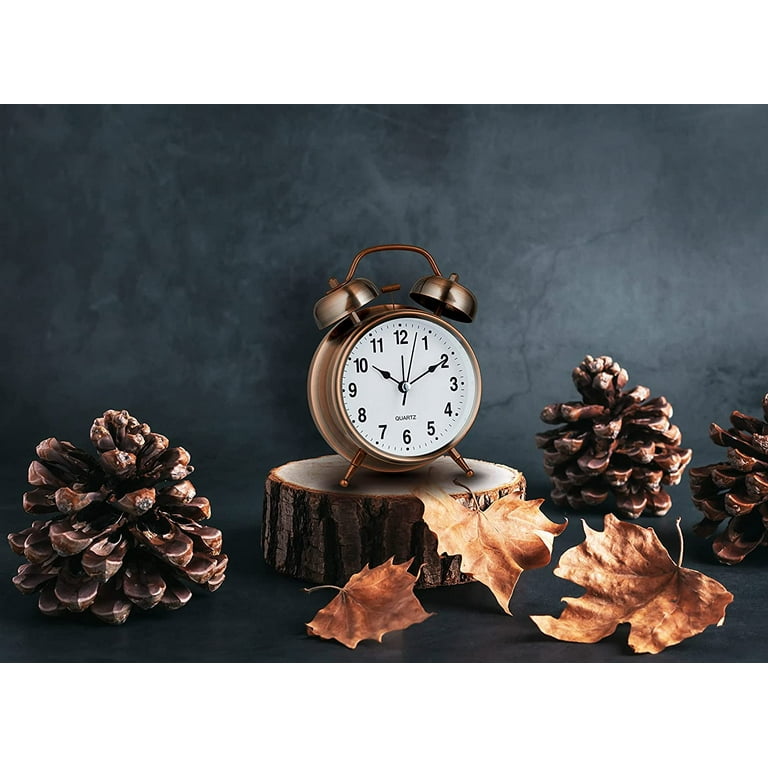The image evokes a nostalgic 1950s feel, akin to vintage home photos or jigsaw puzzles. Set against a smoky black and gray background, the centerpiece is an old-fashioned, shiny gold alarm clock perched atop a wooden disc cut from a tree stump. The clock's dual bell design, complete with clappers, suggests a time long past, and its hands point to 10:10, with the second hand just past the 12. Surrounding the clock is a seasonal arrangement of three golden-brown oak leaves and three pine cones. One pine cone lies to the far left, while the other two are on the right, with one partially cut off on the far edge. The overall composition, with its meticulous detailing of the clock and the earthy decorations, exudes an autumnal charm framed by a subtly contrasting dark backdrop.